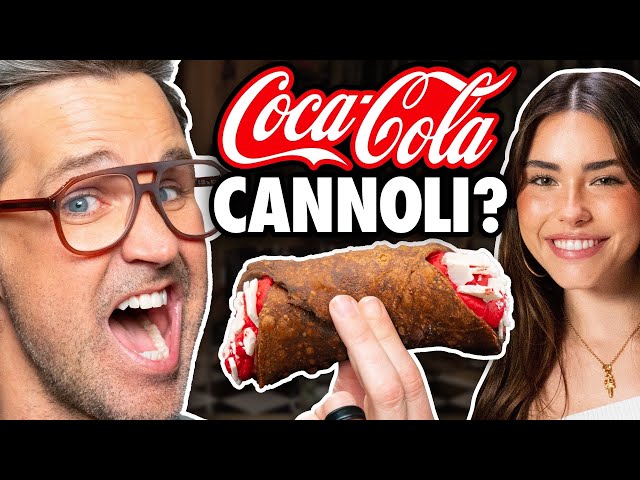Here’s a cleaned-up and detailed caption for the image described:

"A YouTube thumbnail features two individuals highlighting an unexpected culinary experiment. On the left, a white man with brown, thin-rimmed glasses, blue eyes, and a stubby beard holds a cannoli in his right hand. His mouth is open in apparent surprise, and text above the cannoli reads 'Coca-Cola Cannoli?'. On the right, a woman smiles warmly, with pink lipstick, pink blush, and a joyful expression. The unusual twist in the dessert's flavor is designed to capture viewers' curiosity and shock."